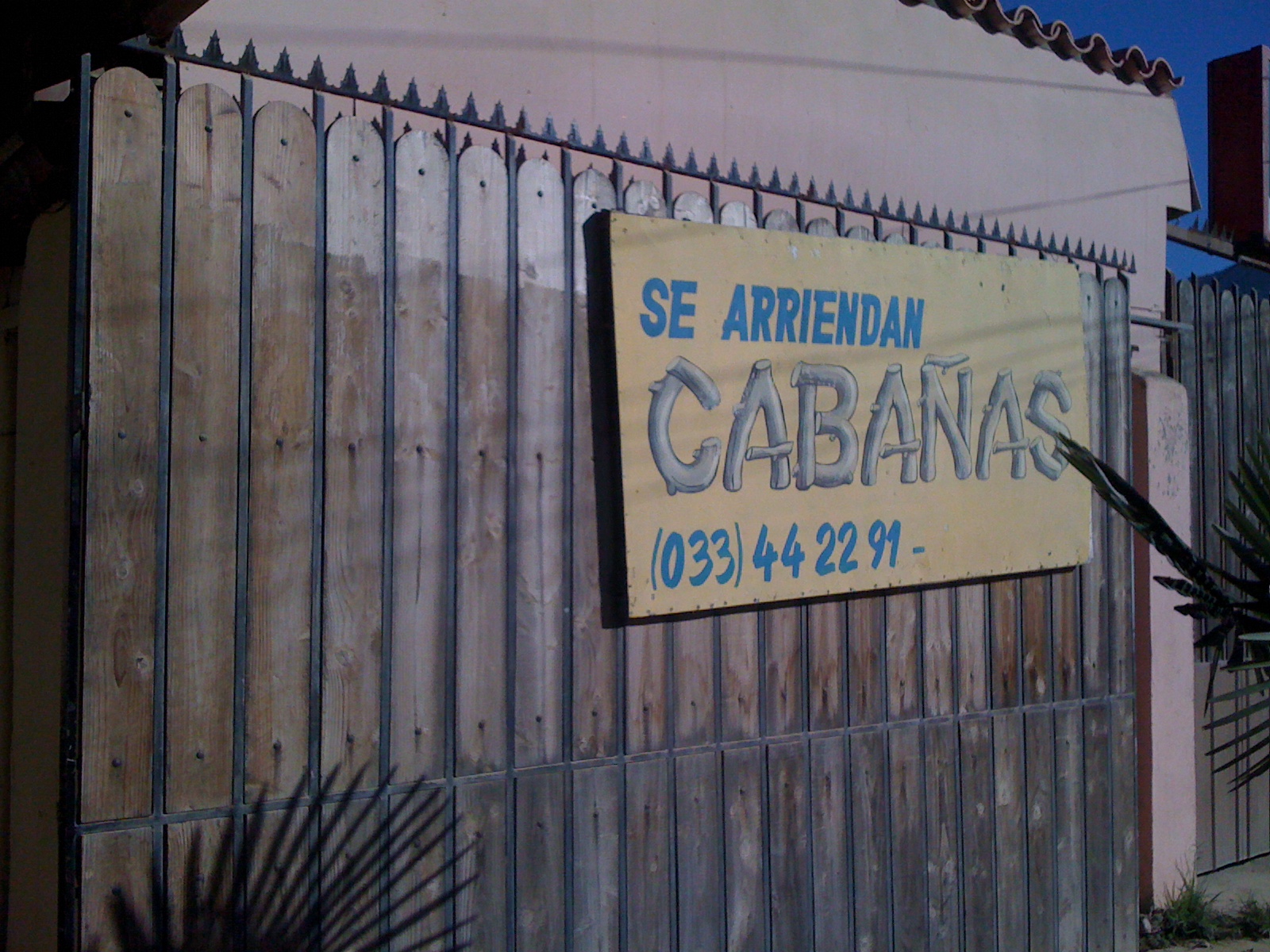This detailed photograph captures a visually captivating scene featuring a black wrought iron and wooden fence with sharp triangular spikes at the top. Affixed to the fence is a slightly tilted, light orange-colored sign with blue and light gray text. The text reads “Se Arriendan Cabañas,” with the word 'Cabañas' styled to resemble pieces of wood, and includes the phone number 033-44-2291. Beyond the fence, the background reveals a light pink stucco-sided building with a unique, wavy-patterned tile roof. The combined elements of the sign and the building create an overall appealing and inviting advertisement for rentable cabanas.